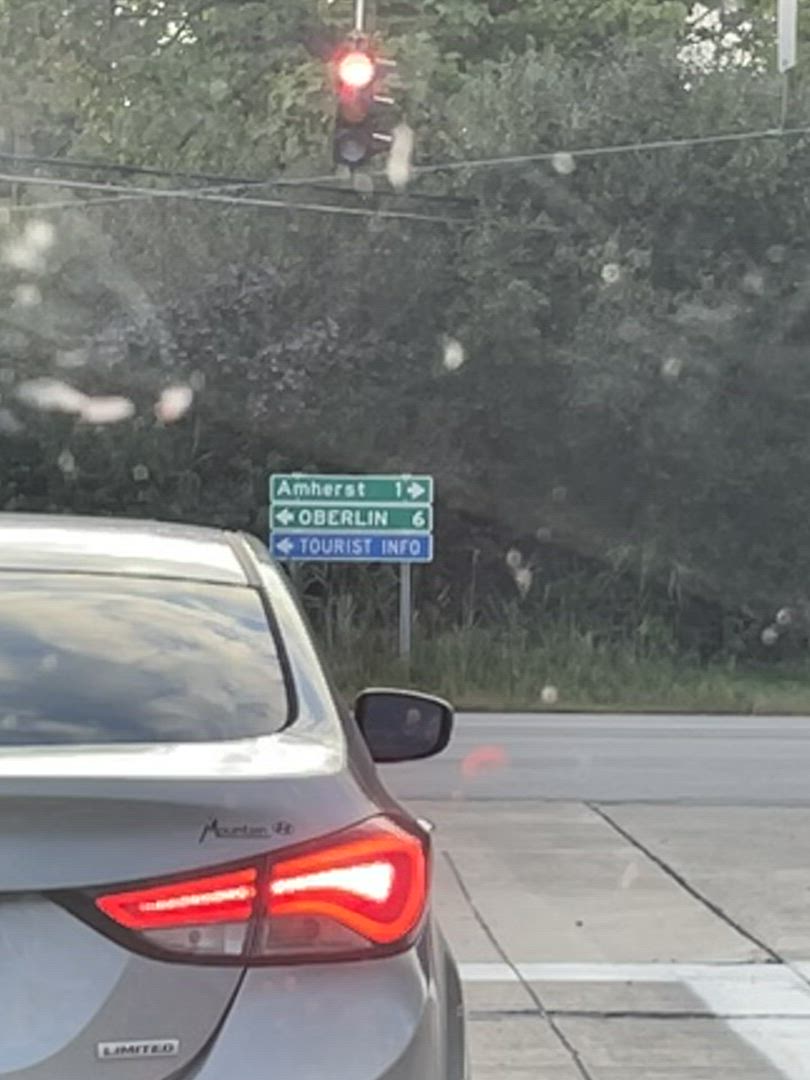The photograph captures an outdoor scene taken from inside a car, possibly through a dirty windshield. In the immediate foreground, there's a silver sedan with its brake lights illuminated, marked with the text "Limited" at the rear. This car is stopped at a red traffic light hovering above the intersection. The intersection appears to be a T-junction, as the road does not continue straight ahead but splits into two directions. On the opposite side of the intersection, lush, overgrown weeds and a backdrop of trees provide a natural barrier. Prominently displayed in the center of the image is a series of directional signs. The top green sign directs to Amherst, one mile to the right, while the middle green sign points to Oberlin, six miles to the left. The lower blue sign indicates Tourist Info to the left. The scene effectively combines elements of nature and road navigation, emphasizing the stillness of the moment at the stoplight.